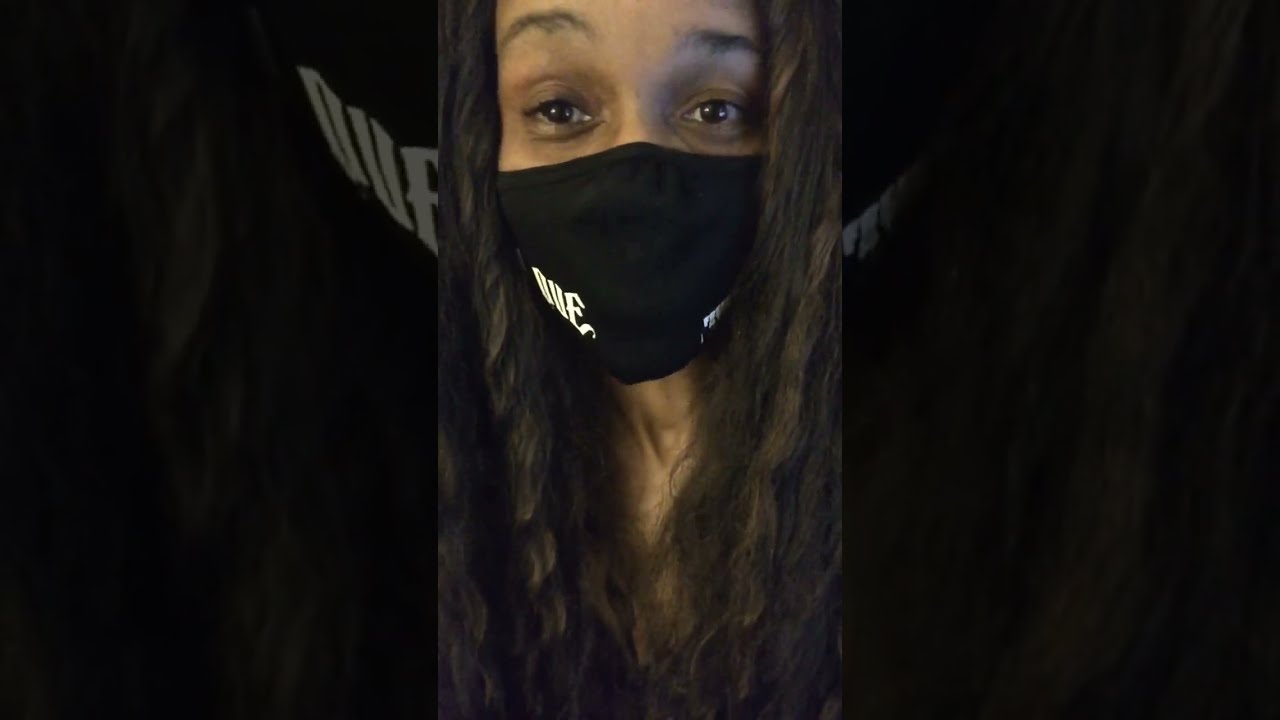The image is a darkened and blown-up photograph of a black woman with very long, wavy brown hair that extends past her collarbone, cascading down on either side of her face. She is wearing a black cloth face mask that covers her nose and mouth, extending down past her chin. On each side of the mask, there are enigmatic white letters, though partially obscured, appear to say "O-U-E" or similar, in gothic font. Her dark brown eyes are wide open, and her raised eyebrows suggest a sense of fear or anxiety. The portrait is zoomed in, filling the frame, and creating an immersive effect where the background appears black, seamlessly integrating with the zoomed-in parts of the mask on both sides. The image starts just above her eyebrows, and her hair partially covers her chest, blocking any view of her clothing.